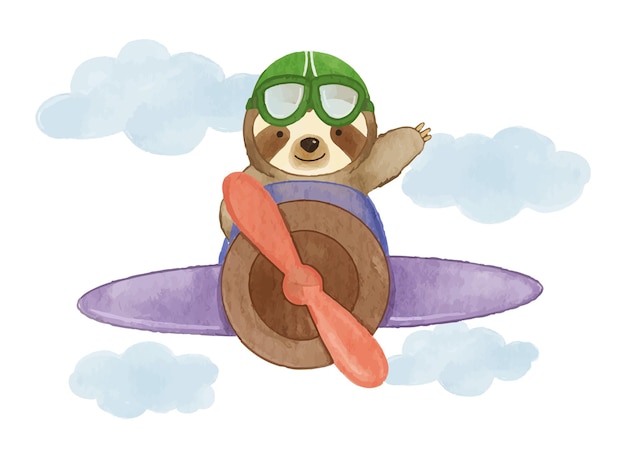In this cartoon artwork, we see a brown bear, possibly a beaver or sloth, sitting in a small airplane with a propeller. The bear has two black dots for eyes and a line for a mouth, giving it a simplistic and charming expression. It wears a green helmet and a pair of green goggles perched on its forehead. One of its hands is lifted in the air as if waving. The airplane is predominantly purple, featuring lilac wings and a distinctive orange-red propeller at the front. The front of the plane also has a brown section highlighted by a light brown circle and a darker middle. The sky is depicted in white with soft blue clouds scattered around, adding a whimsical backdrop. There are clouds to the left and right of the bear, as well as two small clouds positioned under each wing of the airplane.